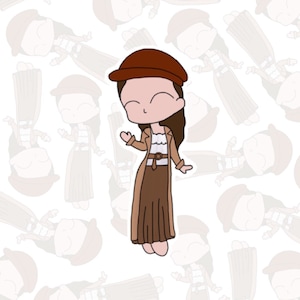The image is a detailed cartoon drawing of a female character with long dark hair and closed eyes, depicted as a girl dancing. She wears a distinctive outfit consisting of a long brown coat, a white blouse with horizontal black stripes, a long brown skirt reaching her ankles, and a brown hat. She has minimal facial features, with just eyebrows and a small line for a nose, and her face is a pinkish-brown color. The character is shown with her right hand upraised as if waving or dancing, and this central figure is vividly colored. The background features numerous faint copies of the same character in various poses on a mostly white, watercolor-like backdrop, creating a unique pattern. The repetition of her image in the background is much lighter and smaller, emphasizing the central, clear drawing.